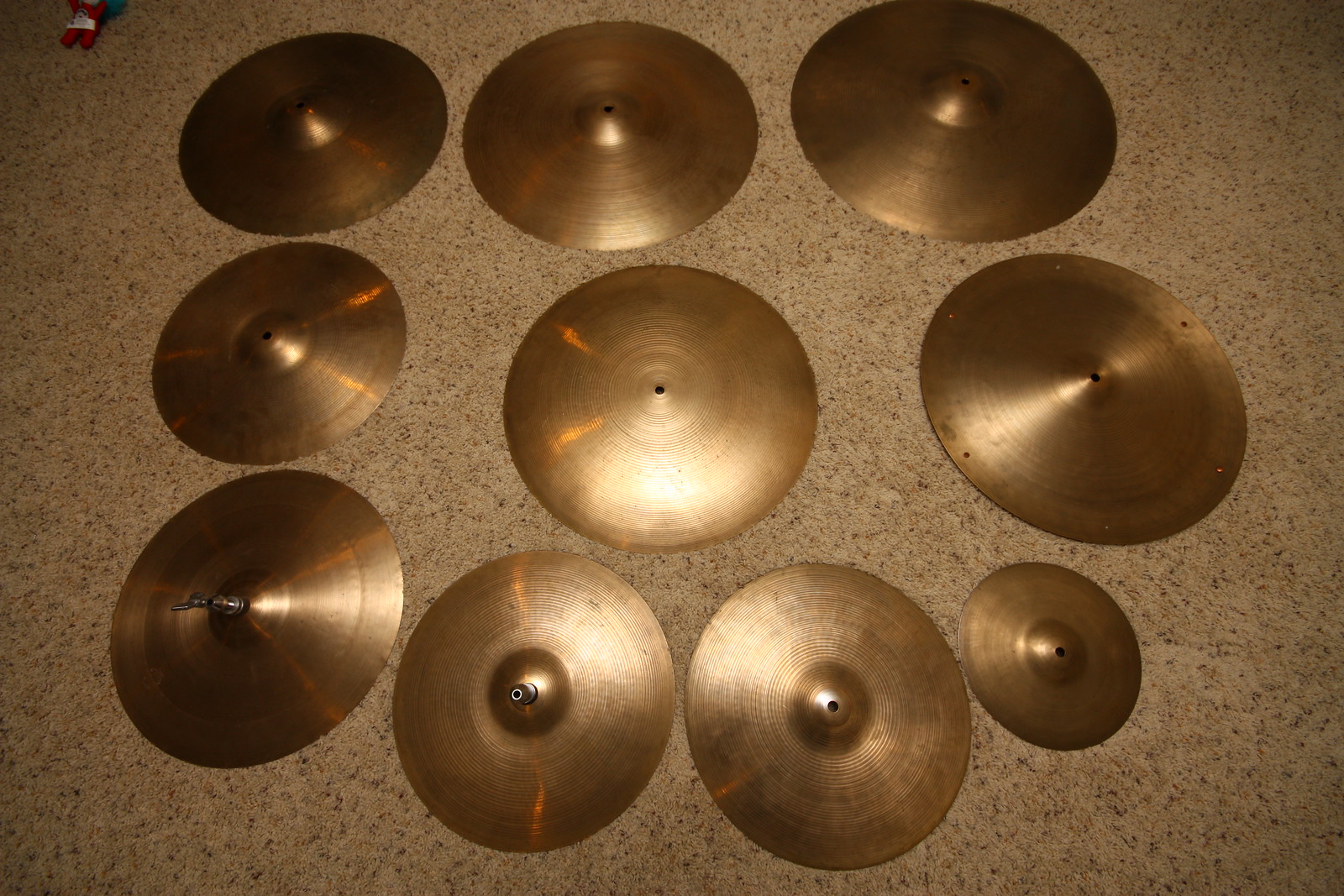An indoor color photograph features a collection of 10 cymbals for a drum kit, arranged on a tan linoleum floor in three rows—three columns with the bottom row containing four cymbals, the smallest one positioned in the lower right. The cymbals are round and brass-colored, appearing more gold due to poor lighting. The set comprises four large cymbals, five medium ones, and one small cymbal. They exhibit signs of use, such as tarnish, especially those on the left and right edges of the image, while the center cymbal appears the brightest. Two of the cymbals still have their tightening pegs attached. The cymbals vary in shape, with some having flat tops and others a small raised dome. The photograph, devoid of any text or branding, suggests an inventory for sale or display purposes.